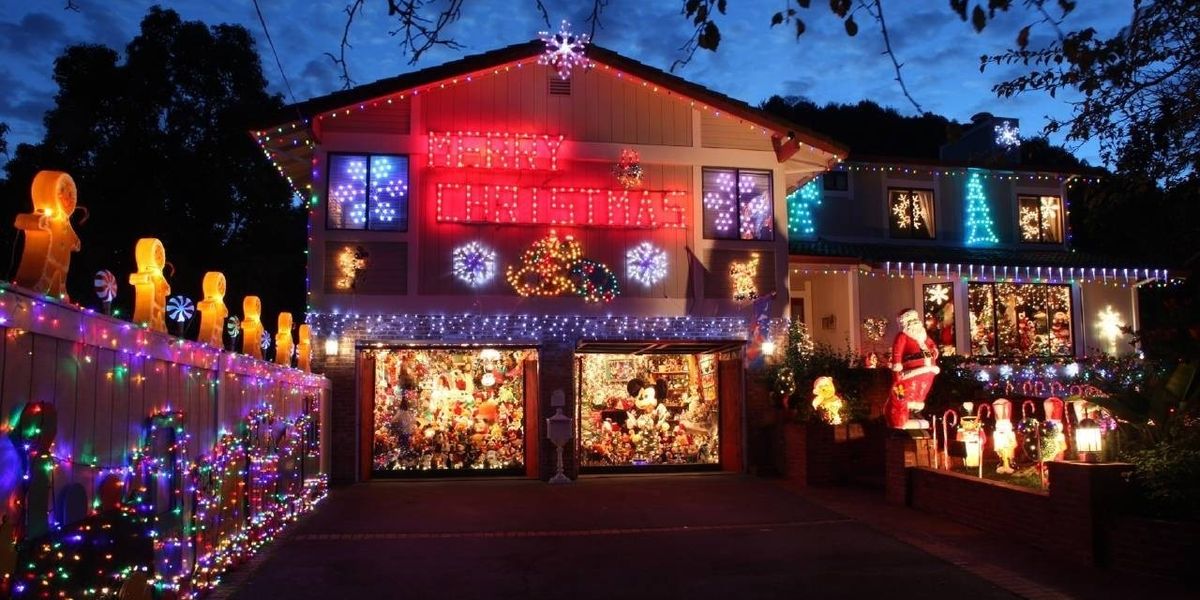As dusk settles over a picturesque two-story A-frame house in the United States, the warm glow of intricate Christmas decorations transforms the home into a festive wonderland. A six-spiked purple star crowns the top peak of the house, setting the scene for the dazzling display below. The main body of the house is adorned with twinkling lights forming the words "Merry Christmas" in red, nestled between two stars—one blue, one purple—and a Santa sled perched above. The windows showcase vibrant light figures, such as snowflakes and Christmas trees, while inside glimpses of toy displays add whimsy to the view. The property’s fence line is equally festive, adorned with gingerbread men and colorful lights. To the right, a statue of Santa Claus in his classic red and white attire stands amidst various holiday dolls, including a prominent Mickey Mouse. This enchanting scene, captured from the sidewalk at twilight with a fading blue sky, epitomizes the joy and exuberance of the holiday season.